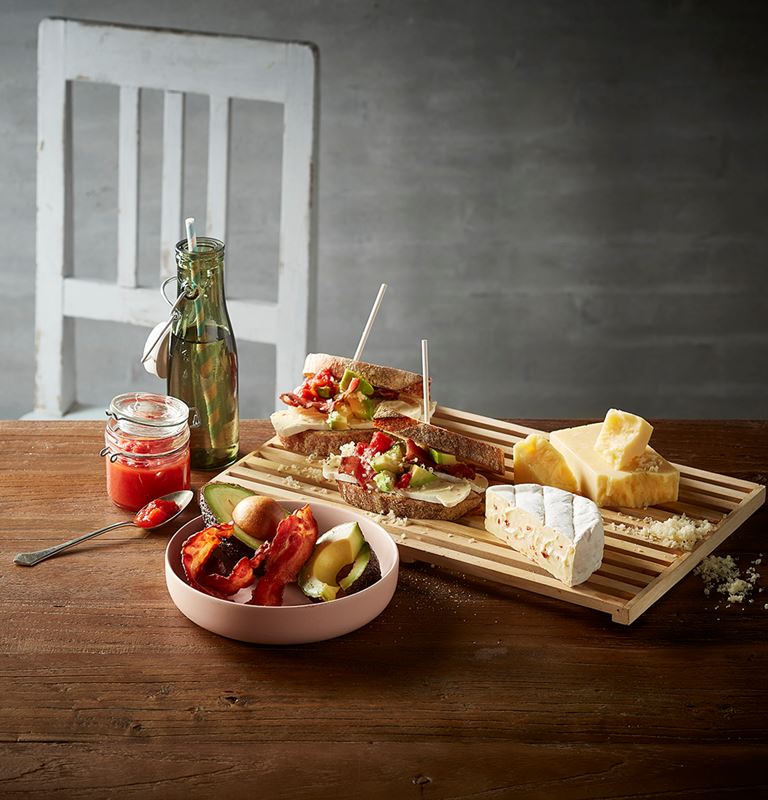This indoor photo showcases a rustic wooden table against a gray stone wall backdrop. A partially visible, chipped white wooden chair adds to the rustic charm. At the center of the table is a tan, light brown wooden cutting board-style platter holding an assortment of cheeses, some of which have shredded bits spilling over onto the table. Two sandwiches, secured with toothpicks, feature tomatoes, avocados, cheese, and bacon. A white bowl contains a mix of avocados and bacon, while a mason jar-style container holds what seems to be jam or jelly, with a spoon dipped into it. A green glass bottle, reminiscent of a Coca-Cola bottle but filled with water, is garnished with a teal and white paper straw. The entire scene captures a cozy, rustic dining setup with a variety of food items arranged in a homely, inviting manner.